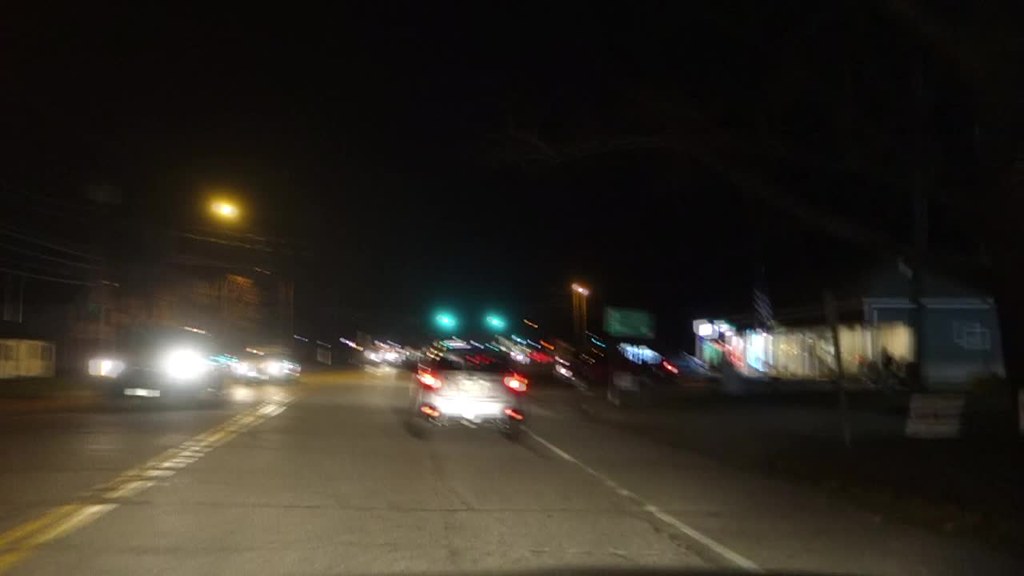A moderately blurry night-time photograph captures a view from inside a moving car, looking down a street. The center of the image prominently features the back of a light-colored car with its tail lights on, positioned in front of the photographer. The car is traveling towards a visible green traffic light a short distance ahead. The road comprises a cracked gray pavement marked by a solid white line to the right and a double yellow line to the left. On the right side of the street, illuminated buildings suggest various businesses, with one noticeably lit up inside and another with parked cars in front. A large green highway sign and street lights emitting halos of light punctuate the scene. To the left, additional buildings can be seen, and headlights from two cars are visible as they travel in the opposite direction, reinforcing the notion that this photograph was likely taken in the United States. A blurred stop sign and the overall hazy effect add to the image's indistinct quality, further softened by the light halos from both the street lights and headlights.